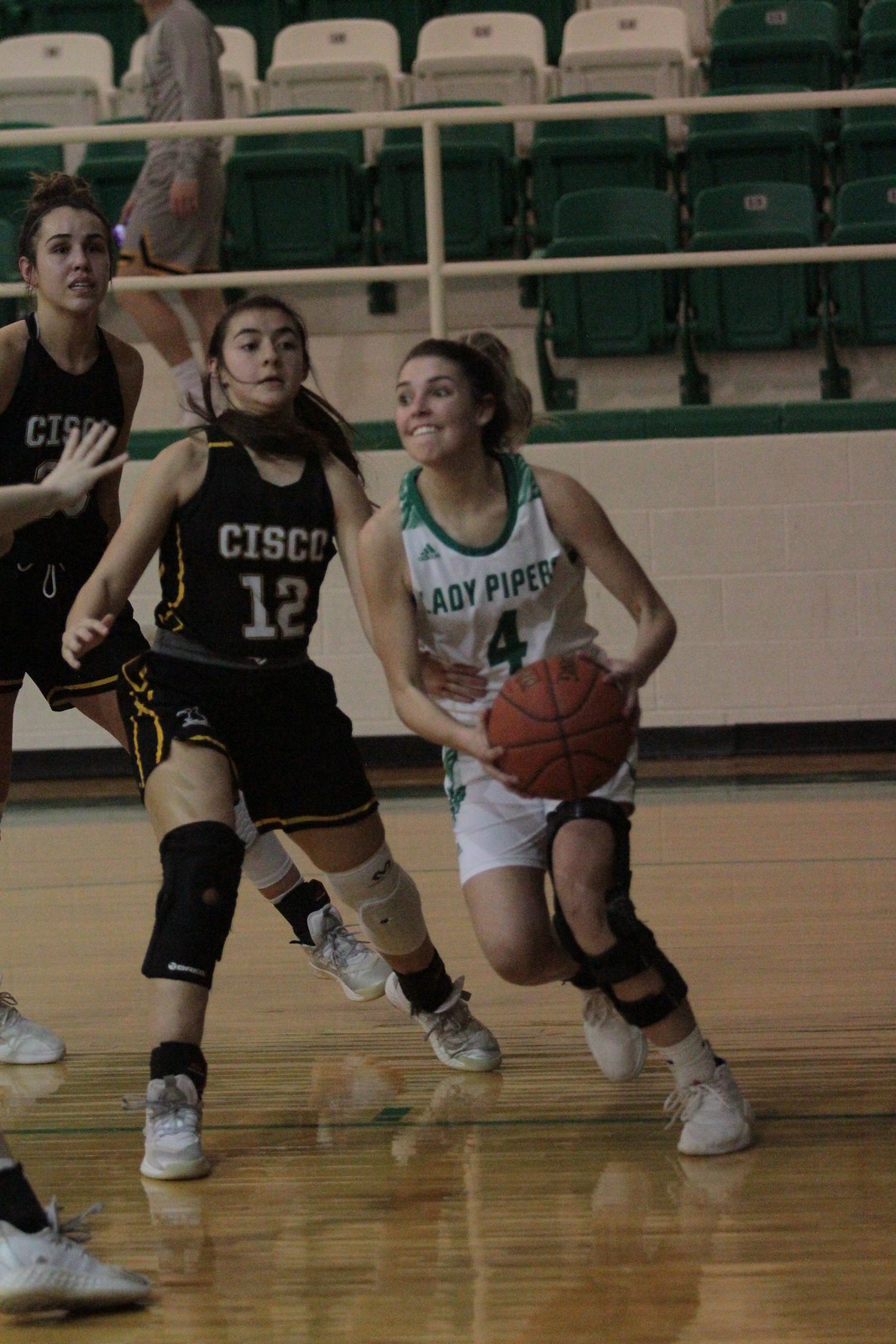In this vibrant action shot of a high school basketball game, three young women dominate the frame, playing with palpable intensity and spirit. The focal point is a determined player from the Lady Pipers, marked by her white uniform with green trim, bearing the number 4. She clutches the basketball with both hands, her face a mix of concentration and exertion as she prepares to make a strategic move. Her knee is supported by a brace, underscoring the physical demands of the sport. 

The two opposing players, dressed in black uniforms with yellow trim from the Cisco team, trail closely behind her, each exuding focus and readiness. Notably, both of them also sport knee supports, signifying the rigorous nature of their play. Behind the players, the stands with a green and cream color scheme are sparsely populated, save for a lone individual dressed in gray walking near the bleachers. The polished floor reflects the intensity of the scene, amplifying the dynamic energy of this high-stakes game.